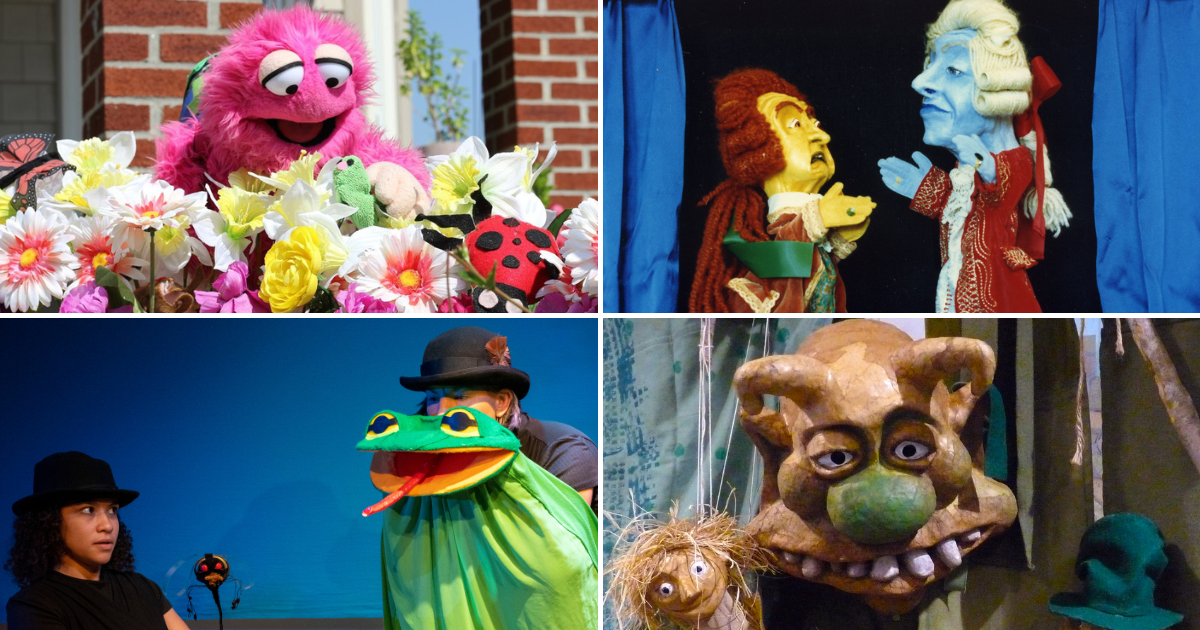This multi-paneled image features a vibrant and whimsical assortment of scenes, likely from a puppet show or a theatrical performance involving puppets.

In the top left panel, a pink puppet with large white eyes and an open-mouth expression gazes down at a colorful array of flowers. The container holding the flowers is cropped out, but the blooms are a mix of yellows, whites, pinks, and reds. Positioned among the flowers are a large black-and-red stuffed ladybug and a similarly colored butterfly adding to the lively scene.

The top right panel showcases two men engaged in conversation, both donning wigs and red robes typical of old-fashioned dress. One man sports a red or brown wig and has light-colored skin, while the other, with blue-colored skin, wears a white wig, adding a whimsical contrast between the characters.

In the bottom left panel, a brown monster figure with large white teeth and a big green nose is featured next to a smaller brown puppet with large white eyes and yellow straw-like hair. The facial expressions on these characters suggest a playful interaction.

Finally, the bottom right panel presents a green frog puppet operated by a man in a black derby hat. Nearby, a woman with dark, long curly hair and a dark-colored fedora looks on with an inquisitive or concerned expression. She wears a dark t-shirt, and behind her is a small black stick figure with a large gray head, white teeth, and red eyes, adding a menacing element to the scene.

This detailed collection of panels captures a lively blend of characters and emotions, evoking the whimsical and imaginative spirit of a puppet show.